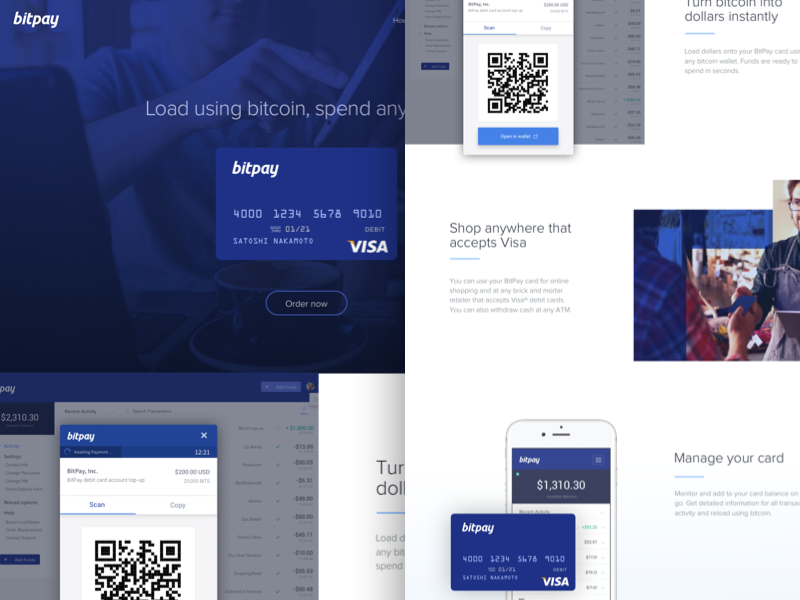The image is a detailed screenshot of a BitPay interface with various elements displayed prominently. The background features a gradient transitioning from lighter blue to darker blue. 

In the upper left-hand corner, "BitPay" is prominently written in bold white text. Approximately six lines down and centered in light blue text, the phrase "Load using Bitcoin, promise, spend any" can be seen. 

Dominating the right side of the screen is a pop-up window with a white background. Within this window, the upper left-hand corner contains a grey box featuring a white rectangle, which holds a scan code at the bottom. The text on the right side, partially cut off, reads, "Turn Bitcoin into dollars instantly," followed by a brief descriptive paragraph.

Below the central text, an image of a royal blue credit card is displayed. This card has "BitPay" in bold white text on the upper left corner and the Visa logo in bold white on the lower right corner, along with various credit card details.

Further down, there is another visual element featuring a square photograph with a blue theme, highlighting the left-front side of a woman's body. To the left of this image, grey text reads, "Shop anywhere that accepts Visa," followed by a light grey paragraph blurb.

Positioned below is an image of a cell phone screen displaying a Bitcoin balance of $1,310.30 in grey text. Overlapping this, the Bitcoin credit card image is shown again. To the right of the cell phone image, grey text reads, "Manage your card."

Overall, the screenshot provides comprehensive visual information on how to load and manage Bitcoin with BitPay, featuring clear instructions and multiple graphic elements to aid user understanding.